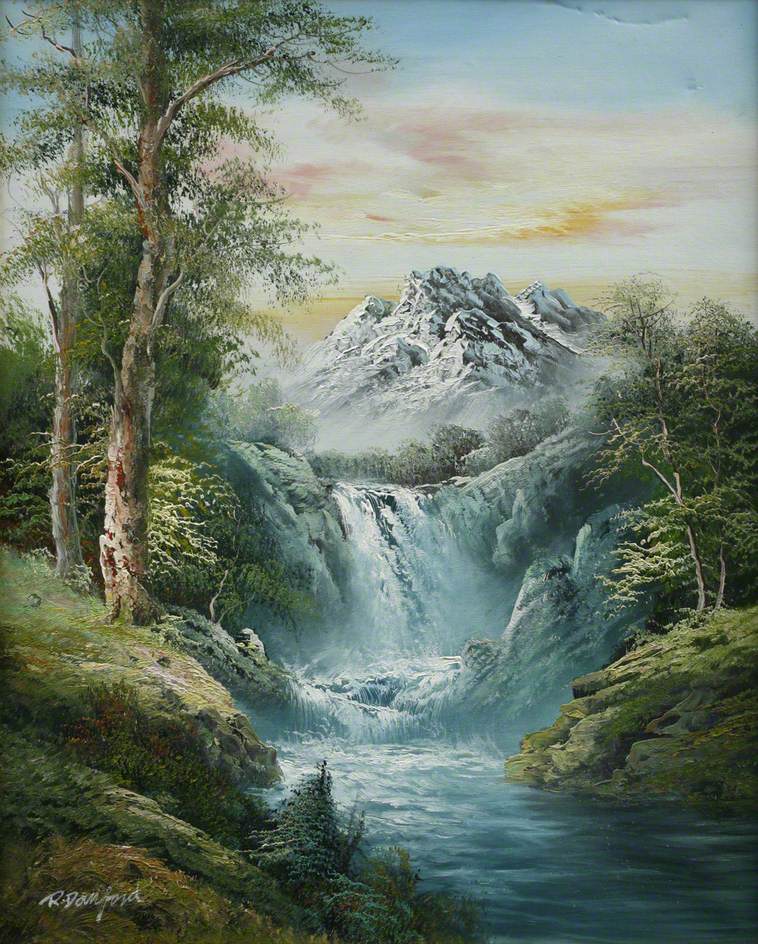This is a detailed painting of a serene natural landscape. Flanking the composition on both the left and right are vibrant green banks adorned with healthy, tall trees sporting lush green leaves, indicative of early spring or summer. Dominating the center is a small, rocky waterfall cascading into a river that meanders through the middle of the scene. The visually captivating background boasts a snow-capped mountain rising majestically, its summit hidden amid streaks of pink and orange clouds, suggesting either dawn or dusk. The sky, transitioning from a clear blue at the top to warm hues near the horizon, adds a tranquil ambiance to the painting. Encircling the waterfall, there is a subtle fog enhancing the ethereal beauty of the scene. A closer inspection of the bottom left corner reveals the artist's signature, possibly reading "R. Damford," skillfully inscribed in cursive.